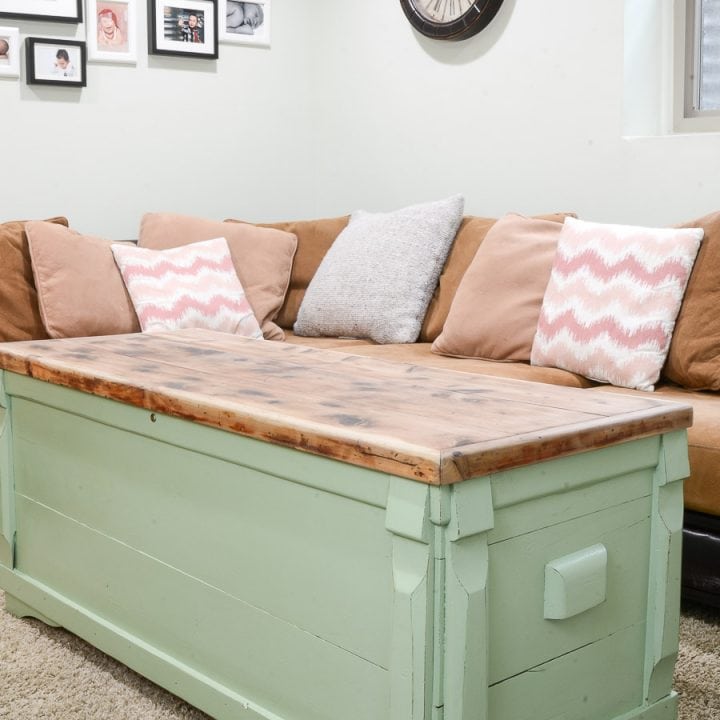The image showcases a cozy sitting area in a corner of what appears to be a living room with white walls. Dominating the area is a tan L-shaped couch adorned with a variety of fluffy pillows. The main pillows are in a matching tan hue, complemented by an array of accent pillows in different colors: three mauve-colored, three pink and white striped, one solid blue, and additional pink pillows with light and dark zigzag patterns. The room features beige carpeting, enhancing its warm and inviting atmosphere.

In front of the sofa rests a prominent coffee table fashioned from an old trunk, with a marbled wood top displaying natural wood grain and a pastel green body. The trunk includes grab handles on either end, though only one is visible. The walls are decorated with framed photos of babies, a partially visible round clock, and a small window letting in daylight. The overall scene suggests a space designed for relaxation and comfort.